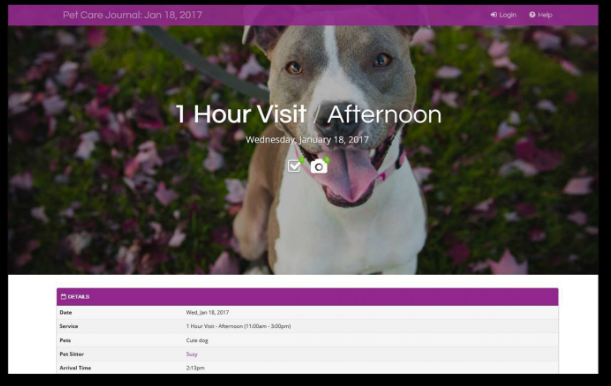The image is a screenshot from a website with a purple banner across the top that reads "Pet Care Journal, January 18, 2017." In the upper right-hand corner, there are options for "Login" and "Help." The main banner features a photo of a dog that is grey, white, and brown, looking directly at the viewer with its mouth open. Overlaying the dog's image is text that states, "One hour visit, afternoon, Wednesday, January 18, 2017." Below this text are icons of a checkmark and a camera.

To the left of the dog, there is a visible leash, and the dog is sitting on grass covered with leaves. Below the main image is a white text box with a purple banner that reads "Details." Underneath this banner, there are labeled fields for "Date," "Services," "Pets," "Pet Sitter," and "Arrival Time." Although these fields are populated with information, the text is small and not entirely legible, arranged neatly in a table format.